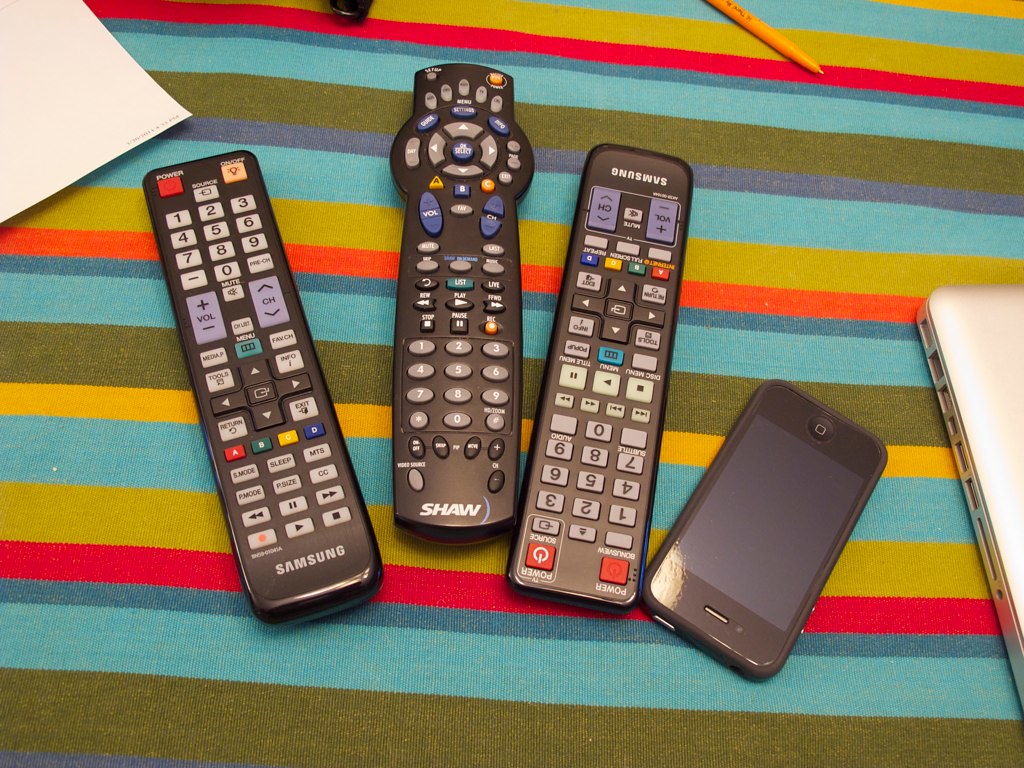On a colorful, multi-striped cloth covering the surface, there are several items meticulously arranged. The striped cloth features bands of dark olive green, light blue, bright red, leaf green, and yellow. Towards the left side of the surface, a white sheet of paper peeks out slightly. Along the top middle, there is a yellowish writing implement that could be a pen or a mechanical pencil. On the right side, the metal edge of a MacBook or another type of laptop is visible. Central to the setup are three distinct remote controls, lined up from left to right. The first remote is a black Samsung with predominantly white buttons and a dark red power button on the top left, along with smaller buttons in red, green, yellow, and blue. The second is a Shaw remote, also black, featuring a long rectangular shape with a circular control area near the top, mostly consisting of gray buttons with white labels. The third remote is another Samsung, closely resembling the first. To the far right of these remotes rests a turned-off iPhone, small, flat, and black. The entire arrangement encapsulates a blend of electronics and writing tools against a vibrant textile backdrop.